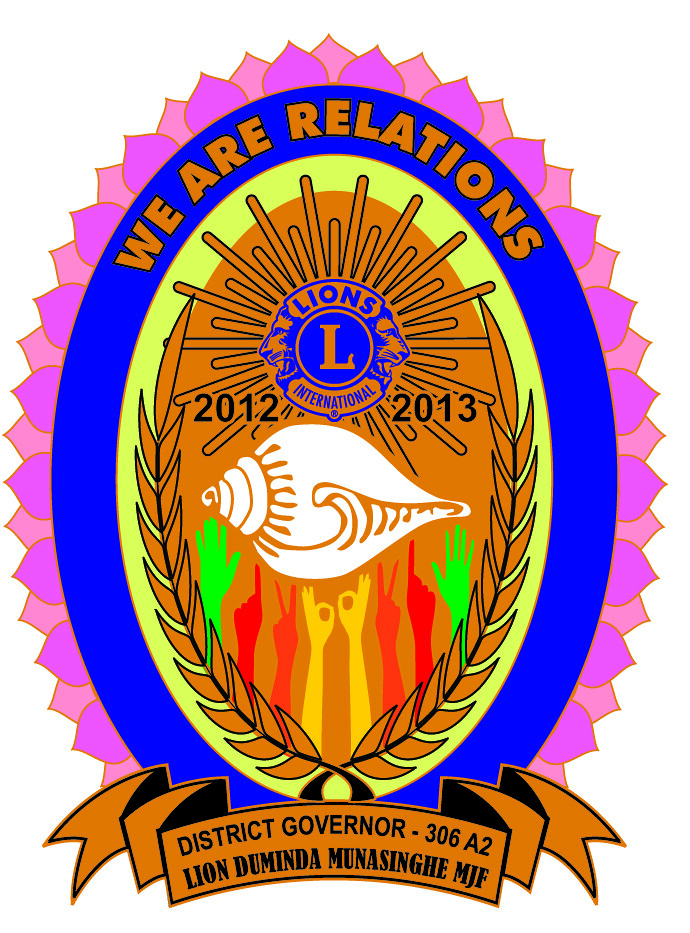The image appears to be a colorful and intricate emblem for the Lions International Club, showcasing the details found in various voice descriptions. The emblem centers around a vertically arranged blue oval, surrounded by pink flower petals. Encircling the oval, a thick purple border bears the golden text, "We Are Relations." Within the oval, there's an elaborate layout featuring multiple elements. 

At the top, the official Lions Club logo is prominently displayed – a gold "L" flanked by two lion profiles, with the words "Lions International" encircling it. Below this emblem, a white seashell is focal, supported by a series of colorful hands in various gestures: green, red, orange, and yellow, arranged symmetrically in both directions, from peace signs to pointing fingers. 

Additionally, the years "2012-2013" are visible on either side of the seashell. Beneath this whimsical display, a decorative scroll reads, "District Governor 306A2, Lion Duminda Muna Singh MJF." The background also includes a medallion-like representation with rays of sunlight and orange laurel leaves, adding to its ornate appearance. The entire design floats without an outer border, resembling a PNG file on a digital flyer or badge.